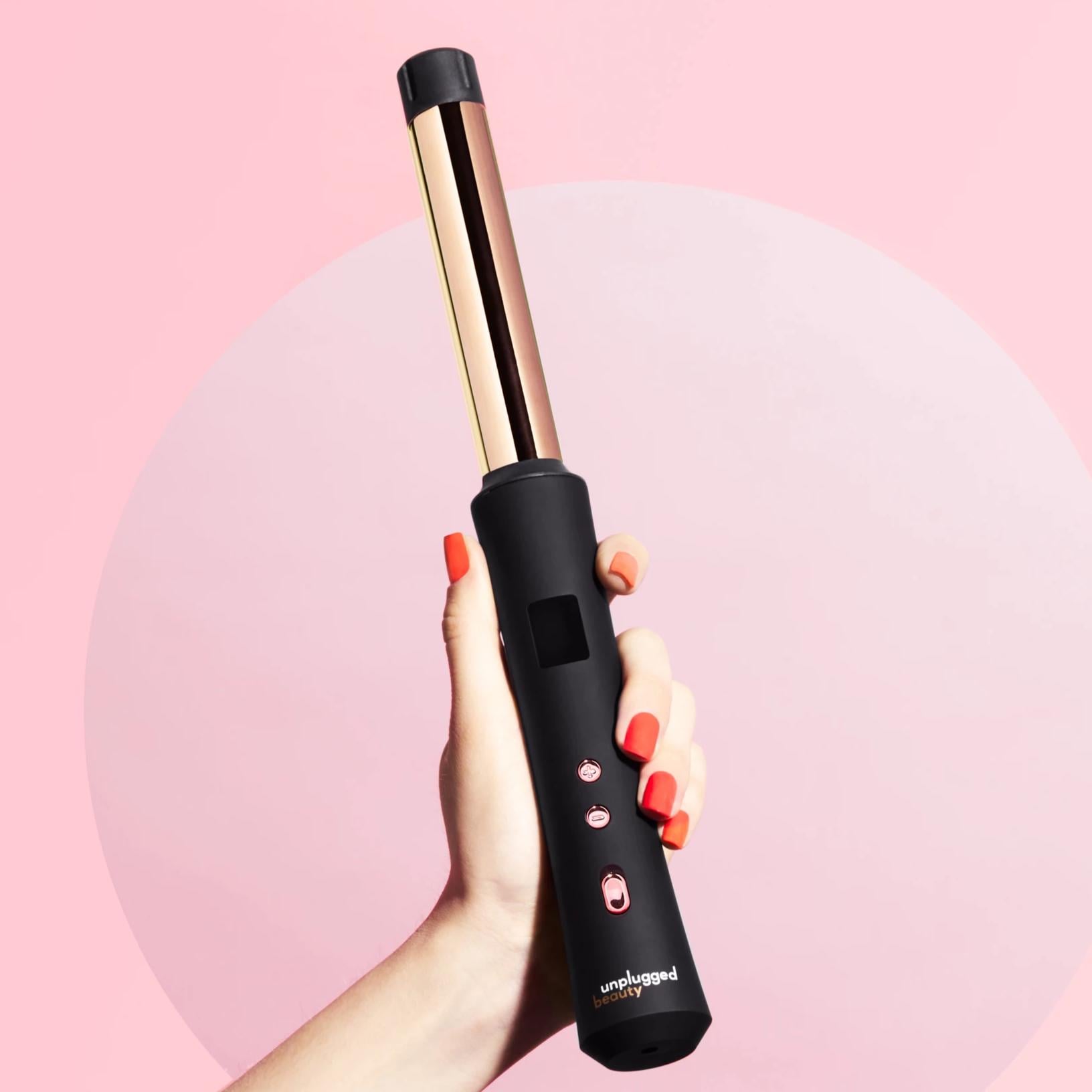In the image, set against a pink background with a lighter pink circle, a Caucasian woman's left hand, adorned with deep red, meticulously manicured nails, gracefully holds a hair appliance. The device, a curling iron, features a gold barrel about one to two inches in diameter, capped with a black rubber tip. The handle is black and accented with three rose gold buttons - two round ones and a smaller switch - likely for controlling the appliance's heat and power. The curling iron is marked with the brand name "Unplugged Beauty," and the entire photograph, with its soft and light color palette, exudes a stylish and modern aesthetic, indicative of a sophisticated marketing campaign.